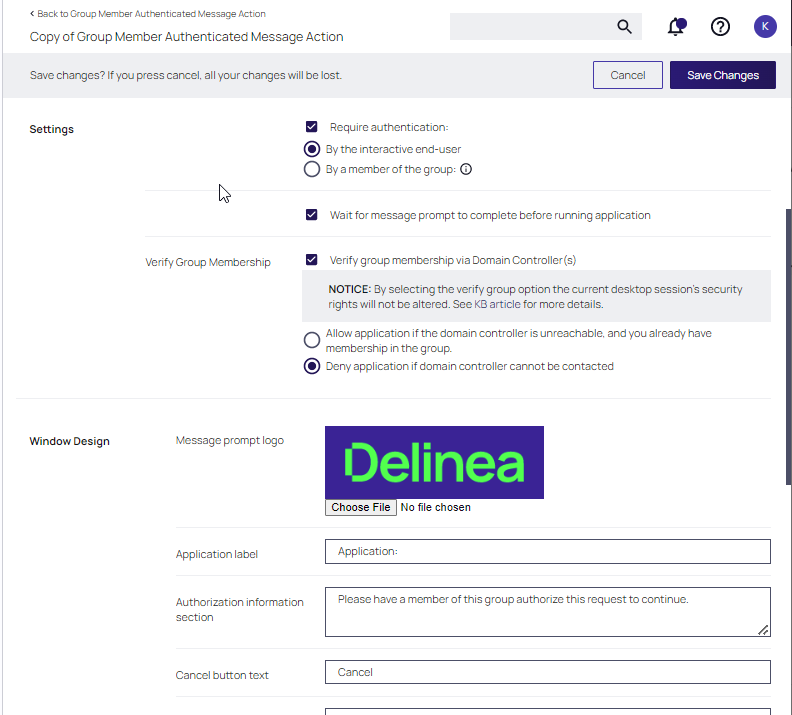This image captures a detailed screenshot of a web application’s settings menu regarding group member authentication messages. At the very top, the interface provides breadcrumbs with the text "Back to Group Member Authentication Message Action" and a duplicate entry below that reads "Copy of Group Member Authentication Message Action." To the right of these, a search field with an accompanying magnifying glass icon is displayed, currently empty. Neighboring the search field are three icons: a notification bell, a question mark, and a blue circle containing a white letter "K."

Directly below this toolbar, a gray bar spans the width of the screen featuring the text "Save Changes." It warns users that pressing "Cancel" will discard all modifications. Both "Cancel" and "Save Changes" buttons are present on this bar for user interaction.

Further down, the section labeled "Settings" appears with various customizable parameters:
- **Require Authentication:** Selected with "Yes."
- **By the Interactive End-User:** Selected with "Yes."
- **By a Member of the Group:** Unselected.
- **Wait for Message Prompt to Complete Before Running Application:** Selected.
- **Verify Group Membership via Domain Controller:** Selected.

Additionally, the interface notes that enabling the "Verify Group Membership" option will alter the current desktop session's security rights and advises the user to refer to the "K8 article" for more details.